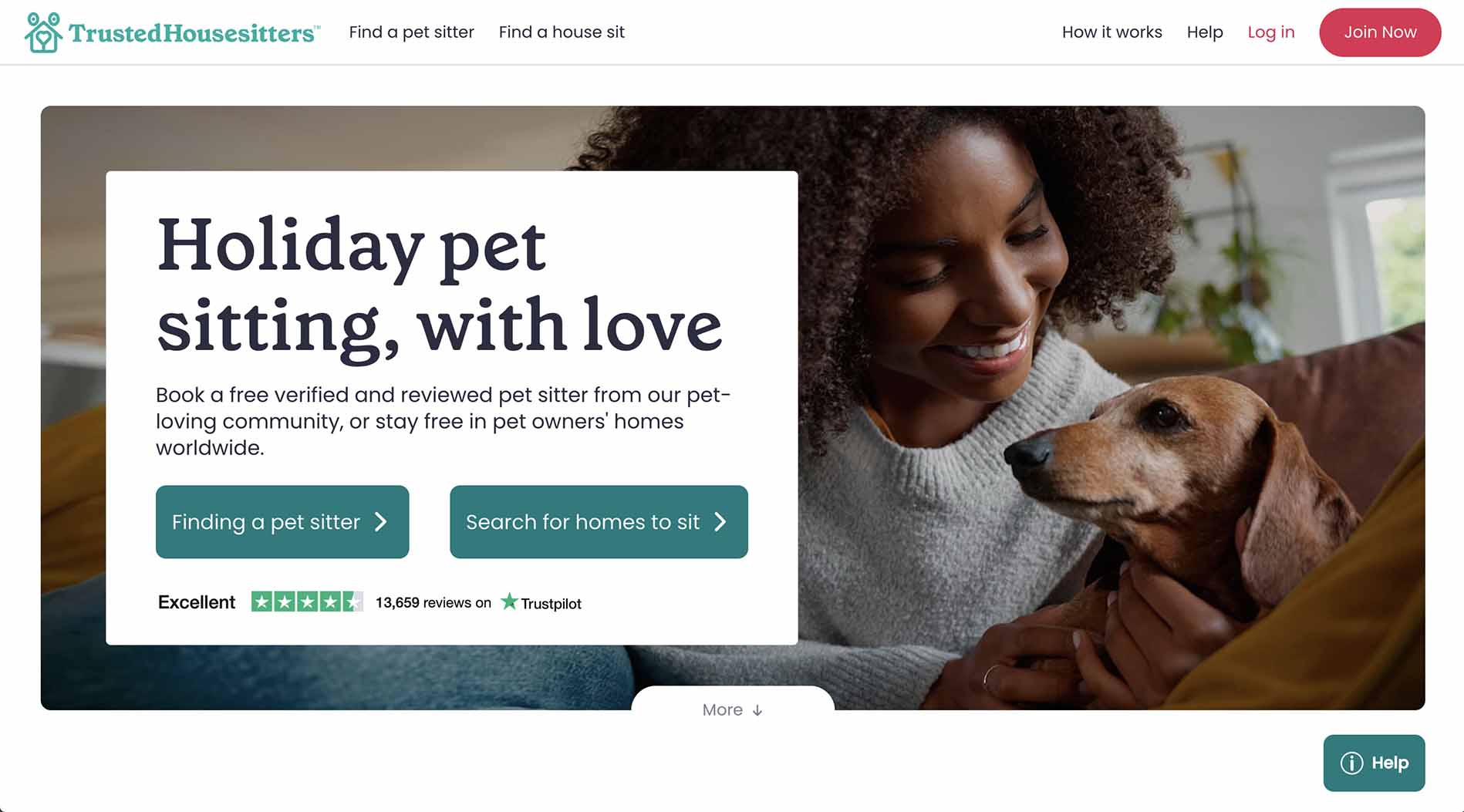The web page for Trusted House Sitters prominently features the company's green business logo in the upper left corner. The navigation menu, presented in black text, includes options such as "Find a Pet Sitter" and "Find a House Sit," clearly indicating the website's purpose of connecting house sitters and pet sitters. To the far right of the menu are additional options: "How It Works," "Help," "Log In" highlighted in red, and "Join Now" inside a red circle.

The central image depicts an African American woman smiling warmly at a brown dog she is holding. The dog is looking to its left. The woman is dressed in a long-sleeved gray sweater and blue jeans.

Beneath the image, within a white information box, the text reads: "Holiday Pet Sitting with Love. Book a free, verified, and reviewed pet sitter from our pet-loving community, or stay free in pet owners' homes worldwide." The options "Finding a Pet Sitter" and "Search for Homes to Sit" are also provided. The site boasts a high Trustpilot rating of four and a half green stars from 13,659 reviews, labeled as "Excellent." There is a tab with "More" and an arrow pointing downwards, suggesting that additional information is accessible with a click.